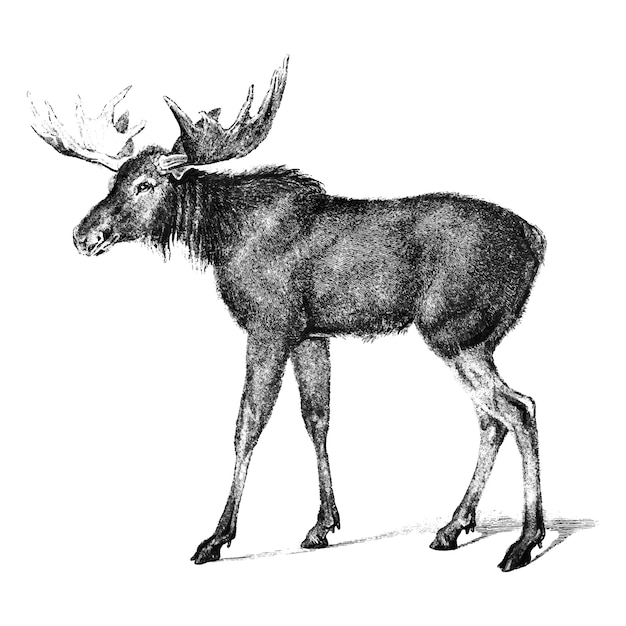This is a detailed side view pencil or charcoal drawing of a young moose, captured in a black and white, hand-drawn style. The moose is depicted facing left, with its head turned slightly towards the viewer, giving a clear view of one of its eyes. Although it has antlers, they are not very large, suggesting that the moose is young, possibly around four years old. The animal appears relatively small and stands on short legs with tiny hooves. Its fur is uneven, with noticeable spots of missing hair. There is no tail visible, and the creature's small face has a subdued expression, almost tired. The drawing features an outline of the moose's shadow cast on a blank white background, emphasizing the absence of any scenery or additional elements. The shading in the drawing is carefully done, capturing the dimensions and form of the moose, especially around the neck, where the shading is deeper and more defined. This meticulous technique lightens across the body, adding to the realistic portrayal of the moose's texture and shape.